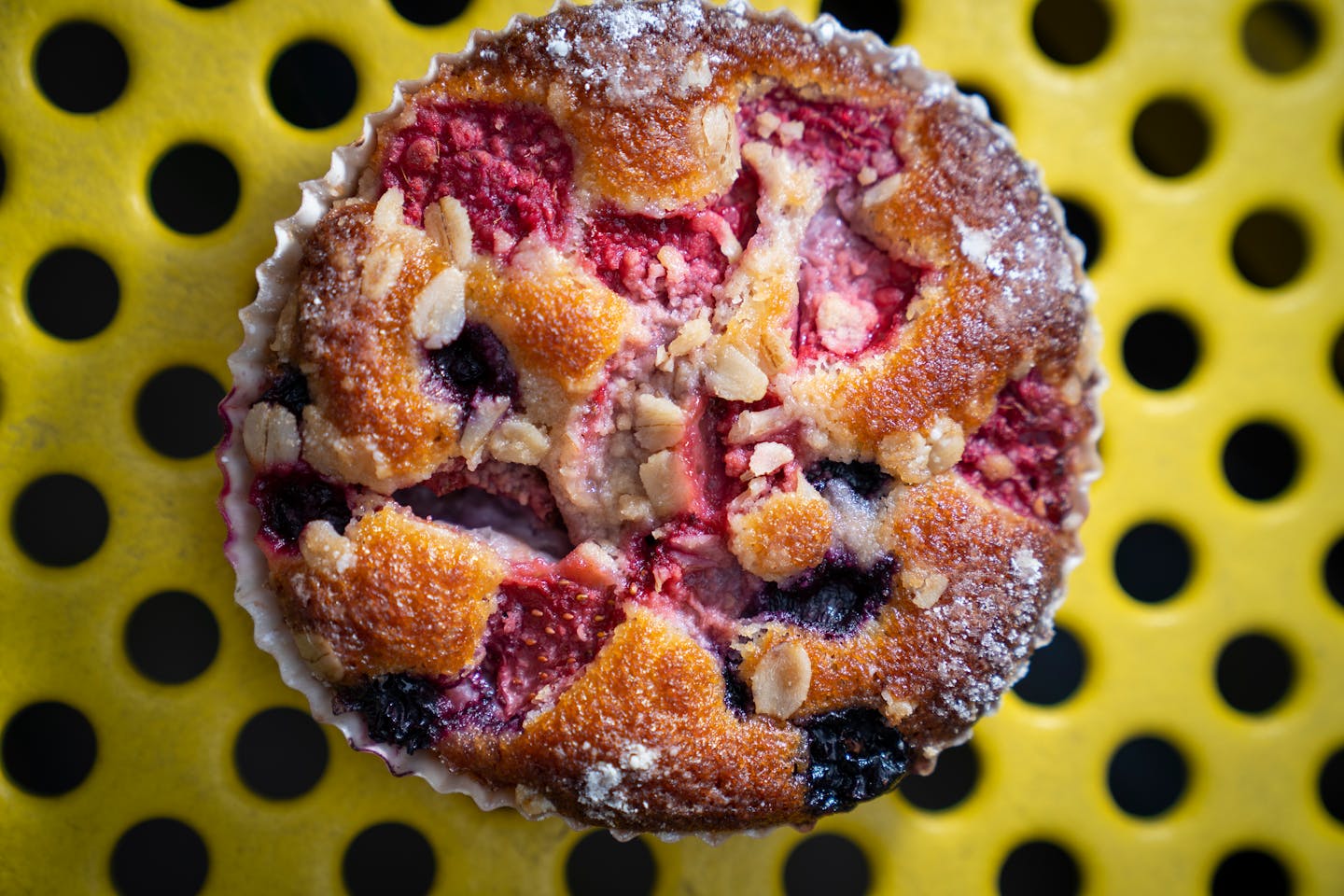This is a high-definition photograph of a freshly baked, mixed-berry muffin viewed from the top. The muffin, characterized by a round shape, features a golden-brown surface adorned with pink and cream hues, particularly concentrated in the middle portion. This mouthwatering treat sports various berries, including blueberries, raspberries, and possibly strawberries, with a delicate sprinkle of oats and sugar on top, adding texture and visual appeal. The muffin is seated in a white cupcake liner, enhancing its inviting appearance. The backdrop is a vivid yellow surface, likely a park bench or picnic table, featuring an array of evenly spaced black holes, adding a structured pattern to the background. The rectangular image is captured in landscape orientation, emphasizing the vivid contrast between the vibrant muffin and the striking yellow-and-black surface beneath it.